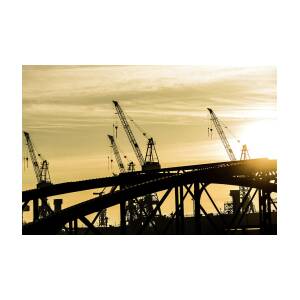The photograph captures a striking industrial landscape at sunset, featuring four towering cranes silhouetted against a dramatic sky. The scene appears to be of an industrial park or a construction site involving a large bridge or monorail structures. The cranes’ towering forms rise into the sky, their cables pulled taut, highlighting the massive scale of the operation. The sky transitions from light bluish-gray to deep orangey-yellow, tinged with wispy clouds, and the sun itself is prominently positioned on the center-right, casting brilliant reflections. In the foreground, the curving arches of the steel structures and scaffolding add depth and complexity, while the overall color palette of black and yellow is interspersed with flashes of white from the sun. The distant view blurs the details, making it hard to discern any human activity, but the grandiosity of the cranes and the ongoing bridge construction stand out as key elements of this captivating sunset scene.